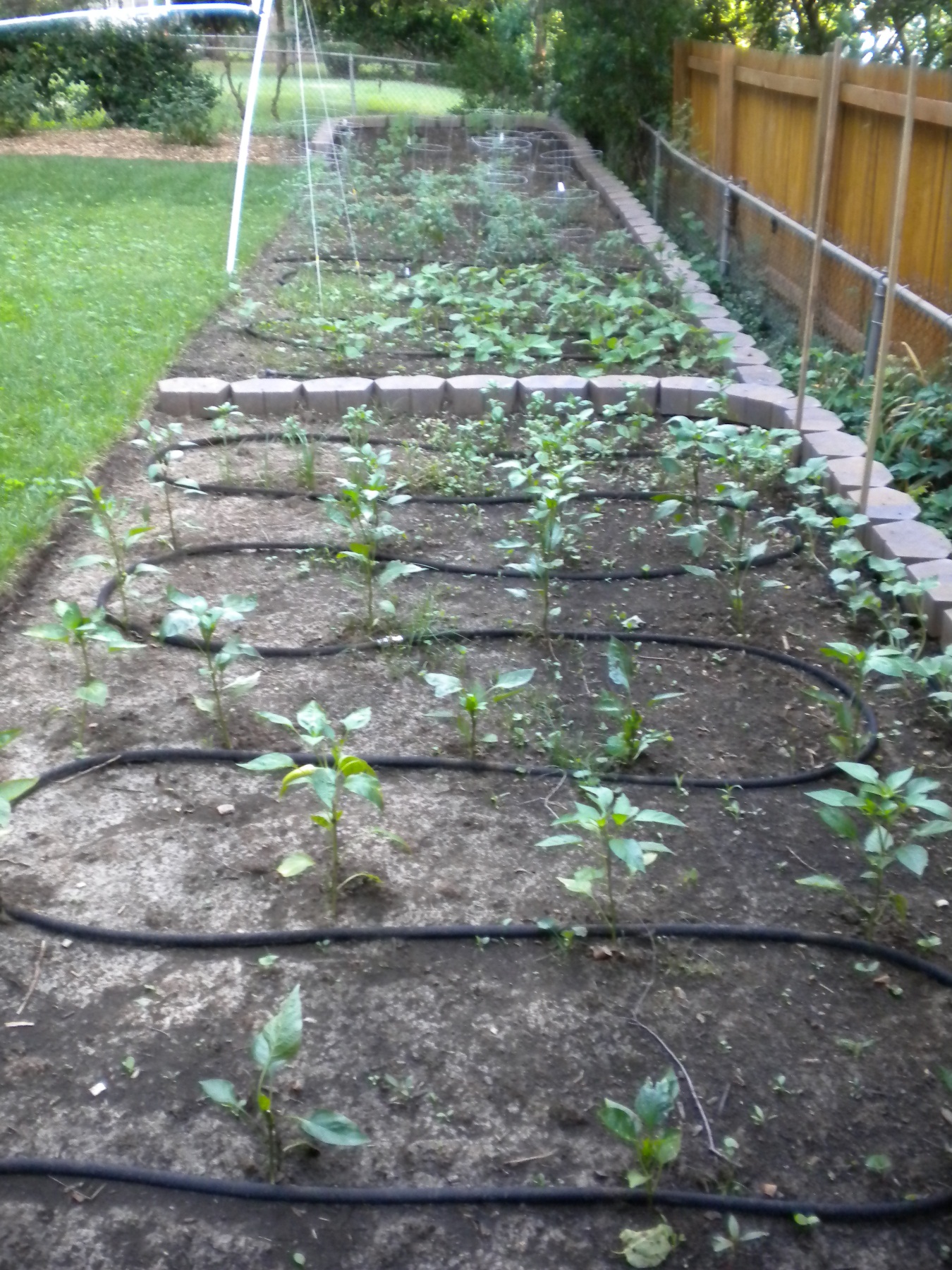The image showcases a meticulously arranged backyard garden, divided into two main rectangular plots filled with rich, brown soil. Each plot contains rows of sprouting plants, standing about six inches tall and spaced five to six inches apart. Snaking through the garden beds is a black soaker hose, ensuring the young plants receive adequate irrigation. The plots are bordered and separated by grey cinder blocks or pavers, adding structure and organization to the garden.

To the right of the garden, a tall, six-foot wooden fence provides privacy, while a metal chain-link fence runs alongside it, offering a dual-layer of enclosure. On the left side, there is a section of well-maintained green grass and neatly trimmed low shrubs with mulch. A white object, possibly a volleyball net or gardening tool, is staked with a white rope on the grass area.

Towards the background of the garden, taller plants, which appear to be tomatoes, are supported by cages, suggesting different stages of growth. In the far back, a mix of green trees and shrubs adds to the lush scenery, completing this picturesque backyard retreat.